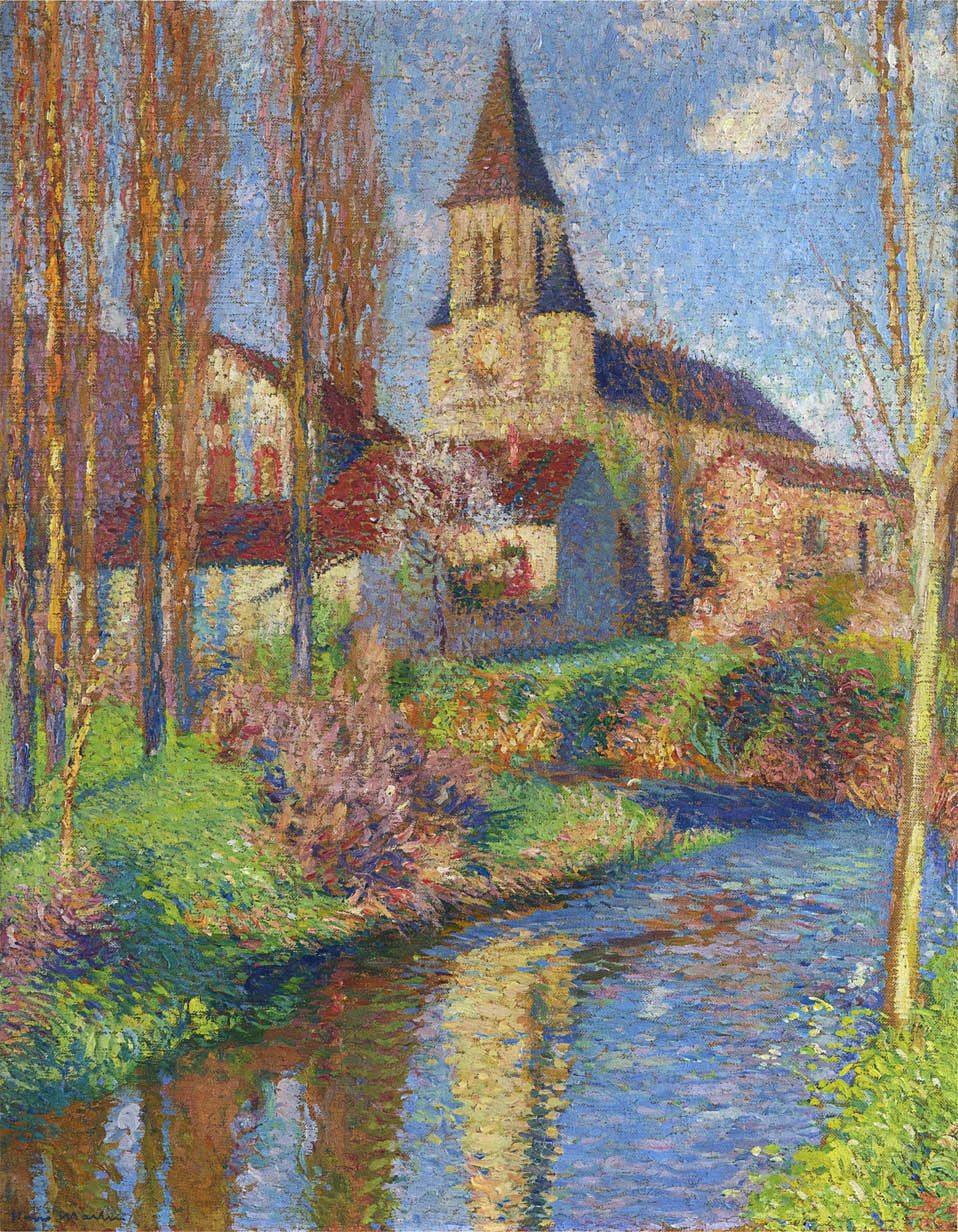This painting, titled "Church and Labistide," exemplifies classic impressionist style, reminiscent of Monet. At the center of the composition stands a large, old-style European church with a white façade and a tower featuring a clock. The church has a prominent spire and a dark, possibly black roof. 

In the foreground, a gently winding blue stream or river runs from the left to the center of the painting. This water body reflects the image of the church, adding depth to the scene. Along its banks, particularly on the left side, vibrant foliage in shades of green, pink, and blue flourishes. 

To the left of the church is a white house with a large shed in front, while to the right lies another structure, seemingly a stone building with a brown roof. Small, colorful houses dot the background, blending softly into the scene. Tall, skinny trees with little to no foliage accentuate the landscape, standing erect on the lush greenery by the river. 

The sky above is a bright, clear blue, scattered with a few indistinct leaves, and the entire painting is characterized by the hallmark of impressionism: soft, blurry edges with bright colors blending together, creating a dreamlike effect.